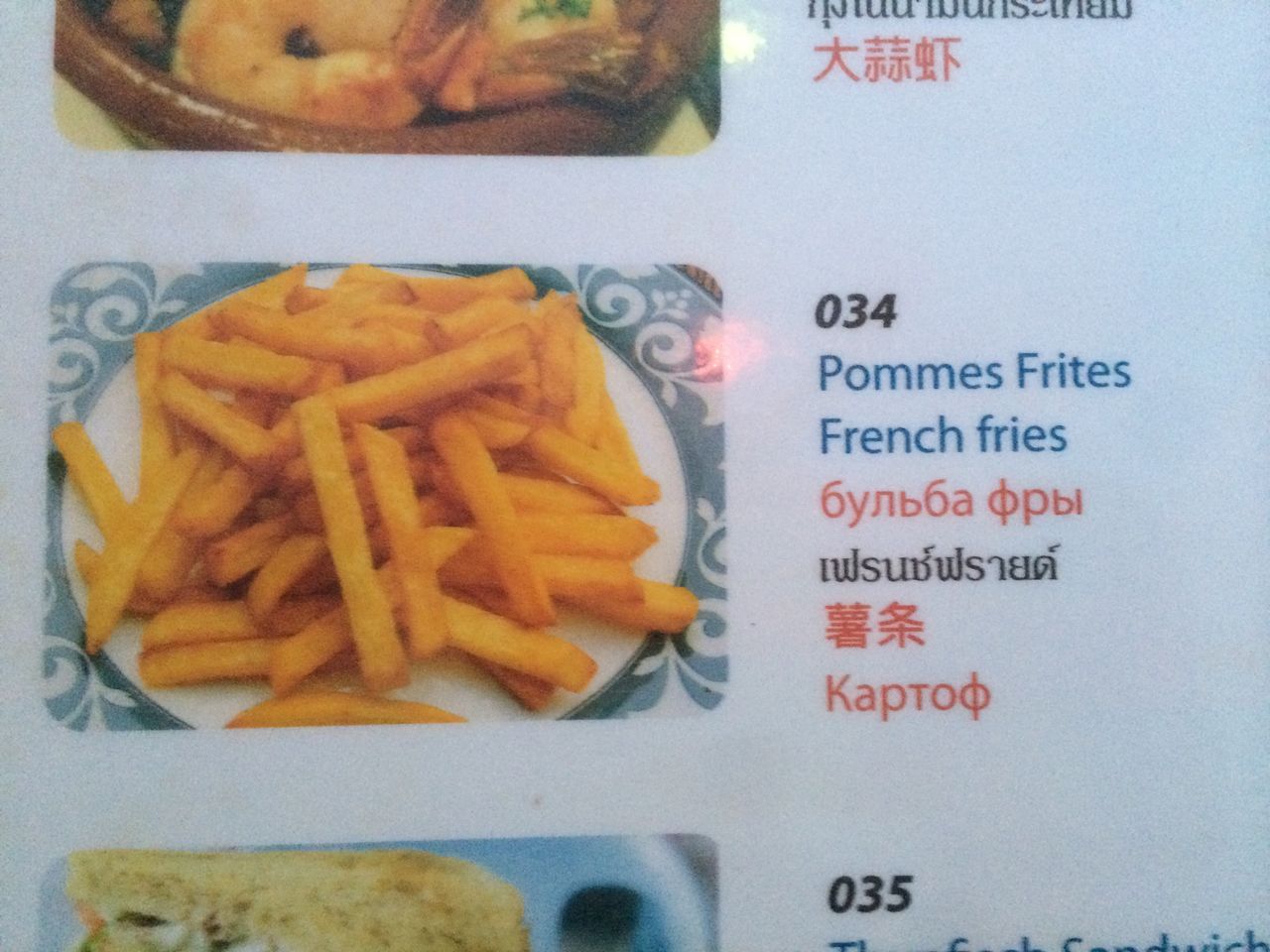The image is a partial shot of a menu encased in what appears to be a clear plastic cover, though it could possibly be framed on a wall. Overhead light reflects slightly on the plastic. The menu background is a pale blue with portions of food photos and text cut off at the top. 

On the left side, a partially visible photo shows a shrimp dish garnished with a sprig of parsley in a brown dish. Above this image is some cut-off black text and a row of shiny red type. Below this, centered and oriented flush left, is a close-up photo of a white plate with a blue border, decorated with white curly tube designs. The plate is heaped with golden-orange French rice. 

To the right of this dish is the number "034" printed in black, followed by the line "blue home wheat cheng" in blue, and then "French rice" also in blue. Below this text is another black line, possibly associated with the shrimp dish.

There is a row of red Chinese characters beneath this, adding a touch of vibrant color. Further down, another row features distinctive characters, including one with a circle and a vertical line, reminiscent of certain European languages. The sequence begins "K-A-T-T-O" followed by the unique character.

Towards the bottom of the shot, there is a small section showing what appears to be the edge of a piece of white toast and the black number "035." The shot is clearly a portion of a larger menu, capturing a mix of textual and visual details.